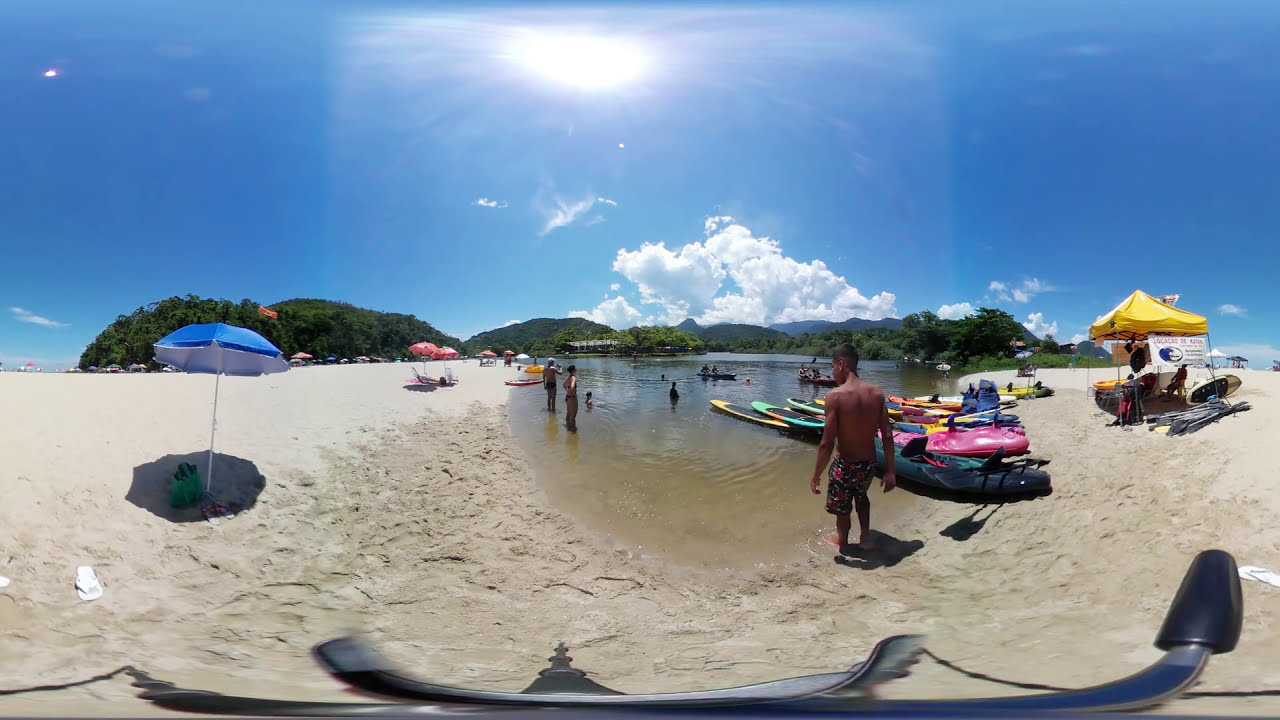The image depicts a lively beach scene bathed in bright mid-afternoon sunlight. The sky is predominantly blue with patches of puffy white clouds, casting a gentle light over the scene. The horizon is dotted with bushy trees and rolling hills silhouetted beneath the cloud cover. The beach is covered in light brown sand, appearing almost white under the sun's rays.

In the foreground, a gentleman in swim shorts stands with his back to the camera, gazing into slightly murky brown water. Next to him, there is a line of paddle boards ready for use. To the right of the paddle boards, a small tent with a yellow roof is set up, providing shade. On the left side of the image, a blue beach umbrella stands prominently, with a green bag underneath it, adding a splash of color to the scene.

The beach appears mildly busy with about 20 people, including men, women, and children, enjoying various activities. Some are seen standing in the water, while others are near the numerous beach umbrellas, with a few red ones scattered about, creating spots of vivid color against the sandy backdrop. The image, free from any text, encapsulates a serene and inviting beach atmosphere, likely situated by a lake rather than an ocean.